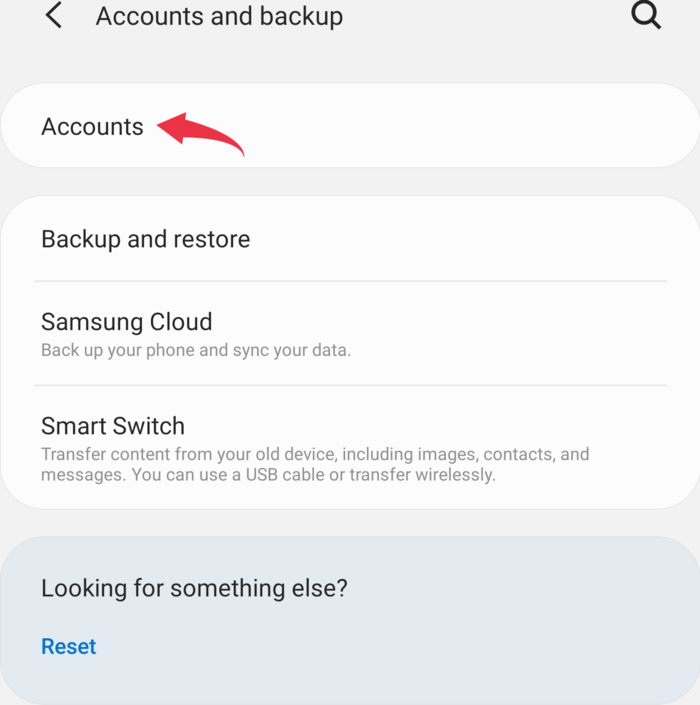This image depicts a screenshot of a smartphone's "Accounts and Backup" settings page. The overall background color is a muted gray, with various sections highlighted in different shades of gray and white. 

At the very top of the screen, the header area displays the label "Accounts and Backup" in bold text. To the left of this text is a left-pointing arrow, and to the right is a search icon represented by a magnifying glass.

Below the header, the first section is titled "Accounts," featuring an arrow pointing towards the text that curves downwards and is highlighted in red, indicating an interactive element.

Following a gap showing the gray background, a new section appears, divided into three parts:
1. "Backup and Restore"
2. "Samsung Cloud" with the subtext "Backup your phone and sync your data"
3. "Smart Switch" with the description "Transfer content from your old device including images, contacts, and messages. You can use a USB cable or transfer wirelessly."

Towards the bottom of the screen, there is a blue rectangle faintly visible in the background. At the bottom-most part of the screen, the text "Looking for something else?" is displayed, followed by a clickable "Reset" option in blue text.